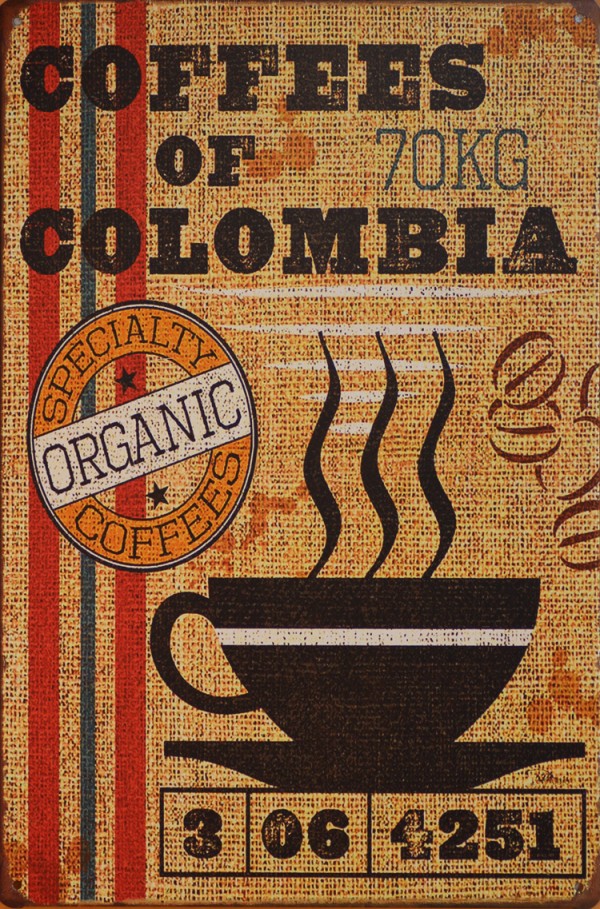The image depicts a rustic and detailed design likely printed on the side of a coffee bean bag. The background has a textured burlap effect with a brown, crosshatch pattern and dark squares at the intersections, enhancing its vintage feel. At the top, the text "Coffees of Columbia" is prominently displayed in black, with "70 kg" written in blue between "Coffees" and "Columbia." Directly below this, the words "specialty organic coffees" are featured, emphasizing their premium quality.

Central to the design is a large, black coffee cup seen largely in silhouette, placed on a matching black saucer. The cup is distinctive with a white stripe across its center and three black steam lines rising from it. There are additional elements, including outlined images of brown coffee beans near the cup. A series of numbers—306-4251—are segmented into separate boxes below the coffee cup illustration, though their significance remains unclear.

Enhancing the visual appeal are outlines of black coffee beans and vertical stripes in red, with a thin blue stripe in between, running down the left side of the text and images, adding a pop of color to the vintage aesthetic.